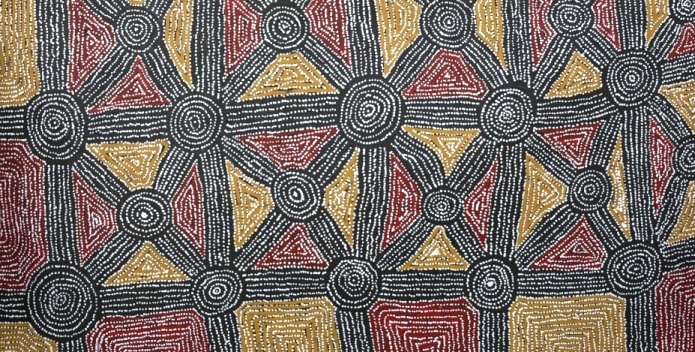The image portrays an intricate, handmade pattern composed of vivid geometric designs and limited colors: black, white, mustard yellow, and cranberry red. The main elements of the design are centered around intersecting lines that form axes, each created with black threads interspersed with white freckles. At the intersections of these lines, detailed concentric circles appear, featuring alternating layers of black and white, culminating in a small white dot at the center.

Throughout the design, horizontal and vertical stripes meet to form squares, and inside each, the pattern intensifies with additional intersecting lines that create X shapes. These lines are further accentuated with smaller white details. The resulting diamond shapes born from these intersections are alternately filled with mustard yellow and cranberry red, each decorated with white dots, adding to the complexity and richness of the pattern.

While the medium is ambiguous—potentially a tapestry, a hand-knitted fabric, or a detailed drawing—the careful and precise execution of the design points to it being a handcrafted piece of artwork. The overall effect is both visually striking and compositionally balanced, highlighting the harmonious interplay of the four primary colors used.